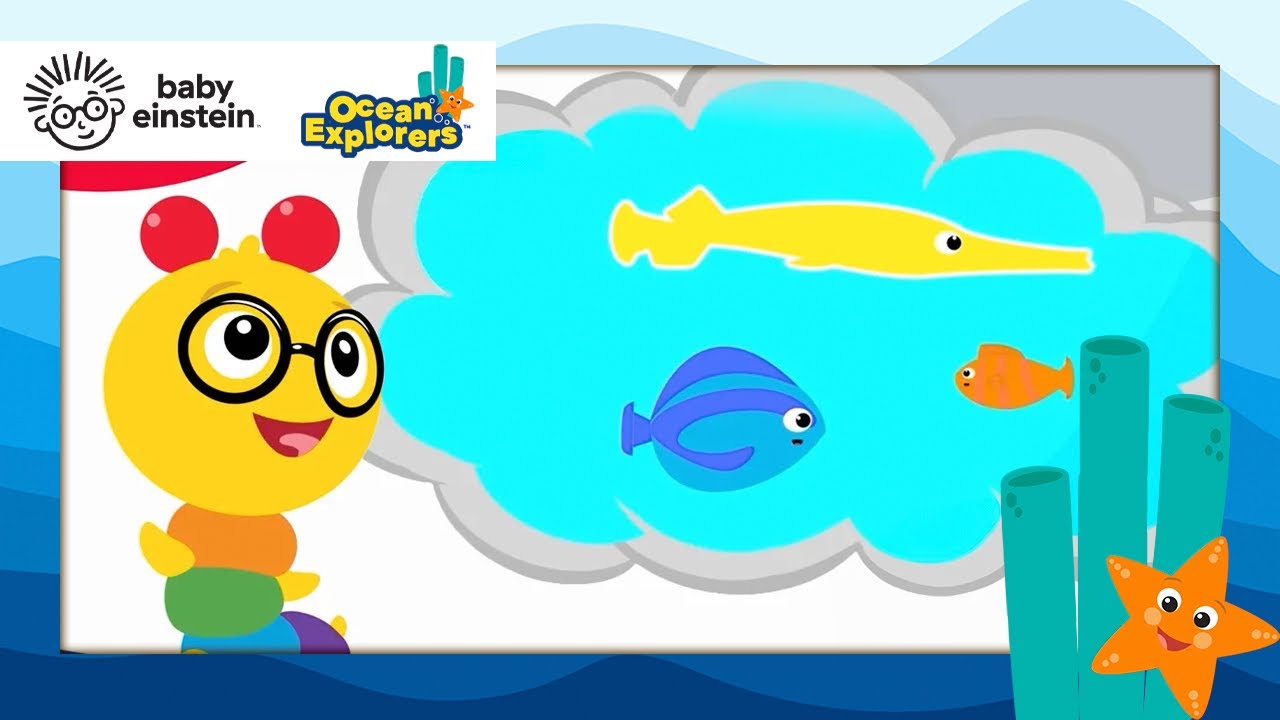This is a colorful advertisement for Baby Einstein featuring a vibrant ocean theme. The top left corner of the image showcases a white banner with the "Baby Einstein" logo, depicting a character with black round glasses, accompanied by the text "Ocean Explorers" in yellow cartoony font. The main frame of the image transitions from light blue at the top to dark blue at the bottom, resembling ocean waves. In the bottom right corner, an orange starfish with white and black eyes is next to some blue coral. Inside the frame, a yellow-headed caterpillar with a segmented body in orange, green, blue, and purple colors, sporting yellow arms and two red antennae, gazes upward. Above the caterpillar, a thought bubble filled with light blue water features three fish – a long yellow fish, an orange fish, and a dark blue and light blue fish. This child-friendly art piece is designed to capture attention with its bright colors and engaging oceanic elements.